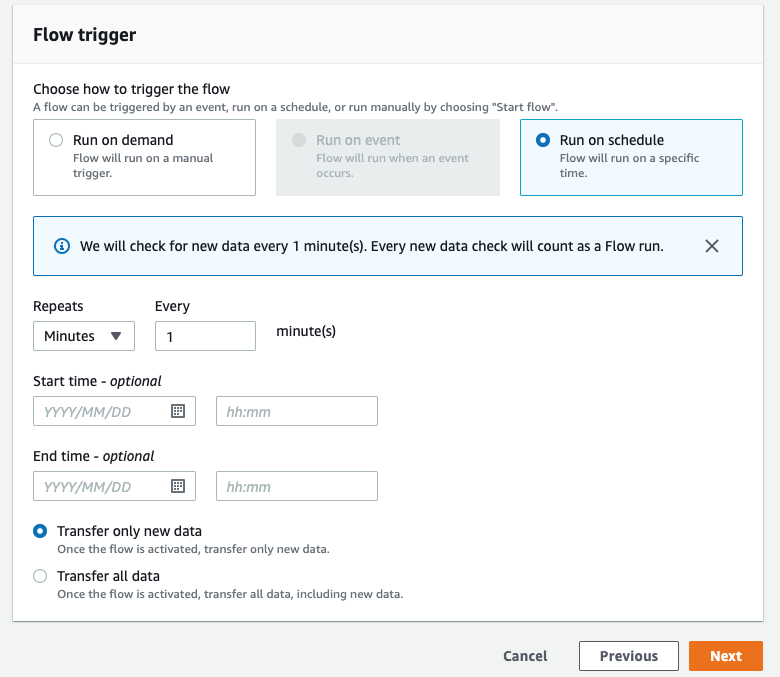This image shows a webpage titled "Flow Trigger" within a browser. The left side of the page features multiple sections, with the main header reading "Choose how to trigger the flow" in black text, accompanied by smaller grey text below it. A detailed explanation follows, stating, "A flow can be triggered by an event, run on a schedule, or run manually by choosing 'Start Flow'." 

Three boxes are presented in a row underneath. The first box, labeled "Run on Demand," is unselected. The second box, "Run on Event," is greyed out and inactive. The third box, "Run on Schedule," is highlighted in blue, indicating it is the currently selected option. Below these boxes, a blue rectangle contains text stating, "We will check for new data every 1 minute. Every new data check will count as a flow run."

Further down, various settings allow for customization:

1. The "Repeats" section has a drop-down menu for selecting intervals in minutes, with "1 minute" currently selected.
2. The "Start Time (Optional)" section includes options to choose a date from a calendar, an hour, and minutes.
3. The "End Time (Optional)" section mirrors the "Start Time" options for date and time selection.

Below these settings are two radio buttons. The first is selected and reads, "Transfer Only New Data." The second option reads, "Transfer All Data."

Outside of the main content box, on the lower right side, are three buttons: "Cancel," "Previous" in a white box, and "Next" in an orange box.